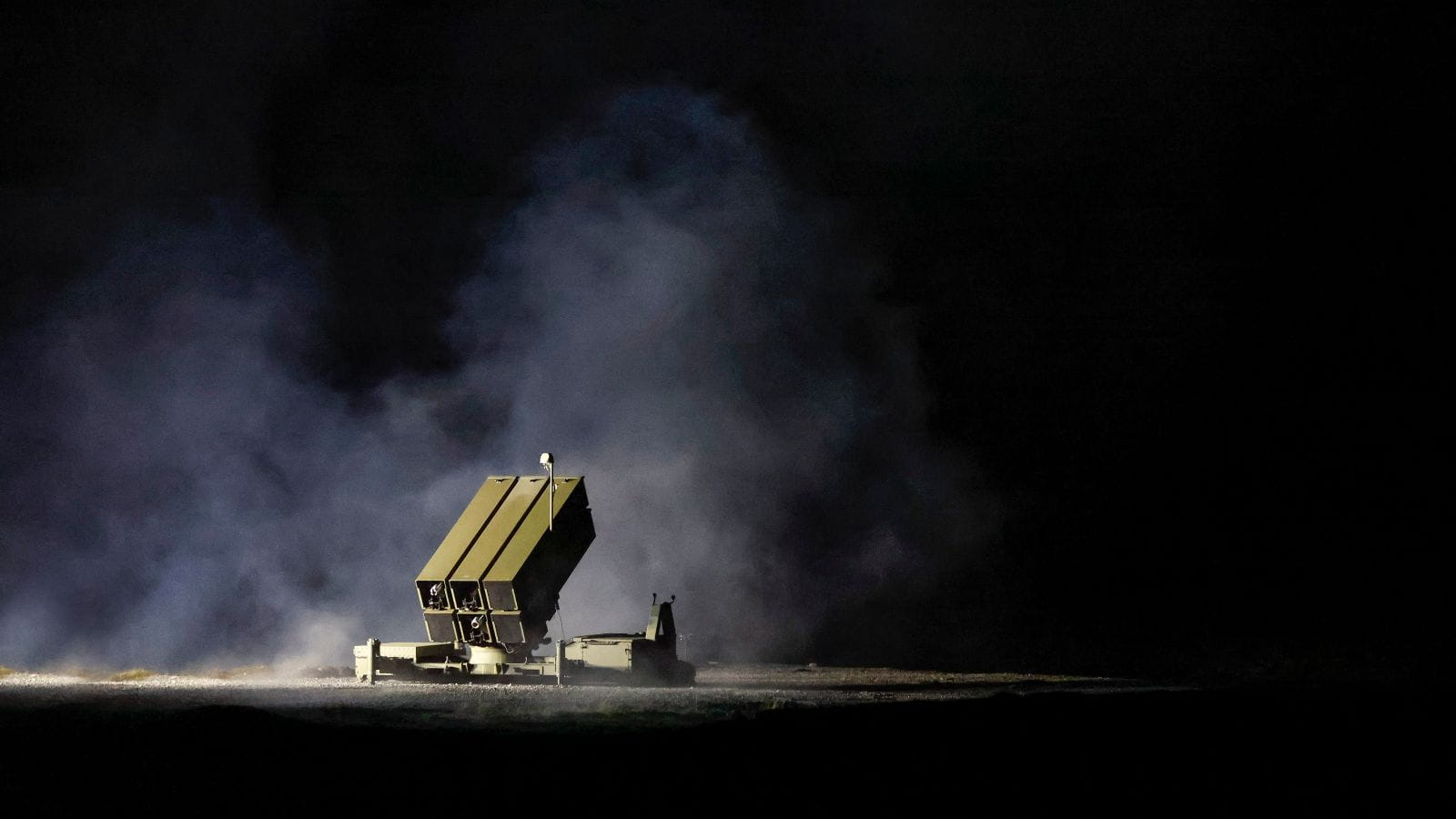In this striking nighttime photograph, we see a mysterious green missile array, composed of six blocky, rectangular chambers arranged together, sitting isolated on barren ground that could be a desert or even a lunar-like surface. The machine is prominently illuminated by a single spotlight, standing out starkly against the pervasive blackness of the sky and the surrounding area, which encompasses almost two-thirds of the frame. There's a notable cloud of smoke or dust hovering around the array, indicating recent activity. Capturing the atmospheric eeriness, the smoke catches and diffuses the light, adding dramatic depth and texture to the scene. The setting's emptiness and the focused light on the missile array give the image a surreal, almost otherworldly feel.